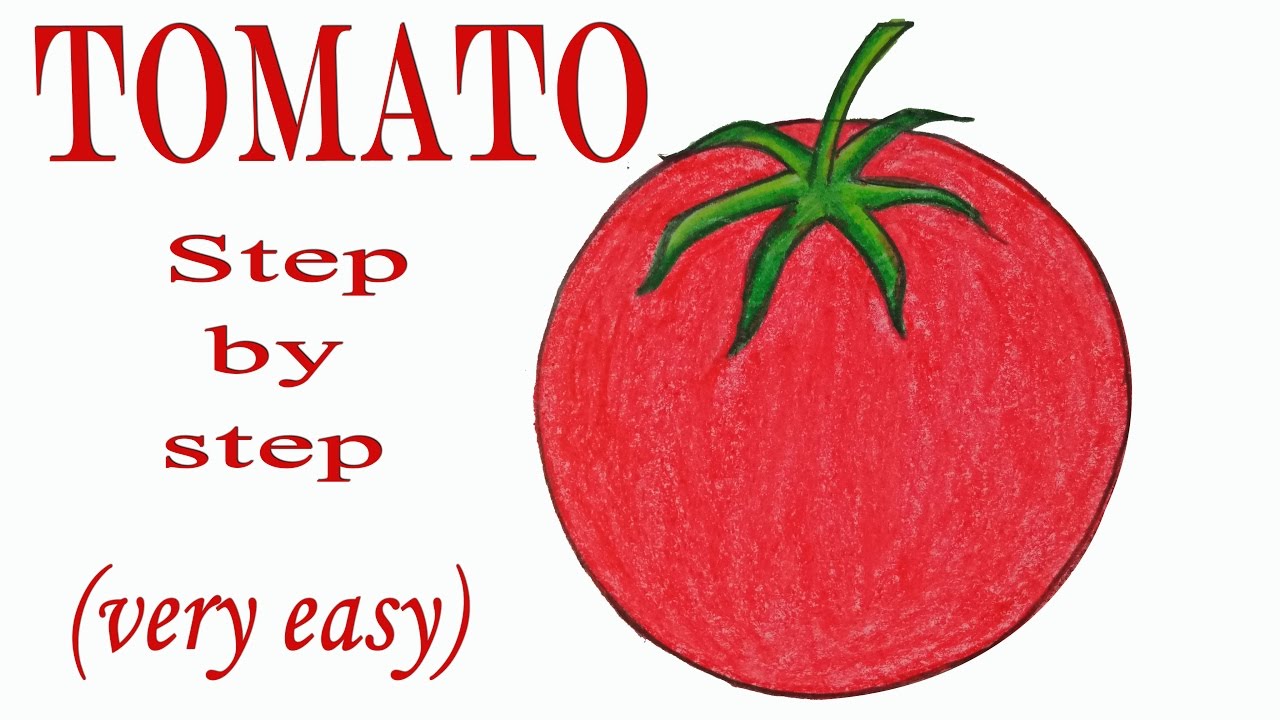This image features a childlike crayon drawing of a large red tomato on a blank white background. The tomato is a simple circular shape with areas of lighter shading, giving it a textured appearance. It has a thin red outline and green leaves at the top with a black outline, and the stem is highlighted with a yellowish-white color. To the left of the tomato, the word "TOMATO" is prominently displayed in large, all-capital red letters. Below this, in laser-printed text with one word per line, it reads "Step by Step." In smaller, italicized lowercase letters, enclosed in parentheses, it says "very easy." The simplistic and vibrant drawing, combined with the straightforward instructional text, suggests an easy-to-follow guide designed for beginners.